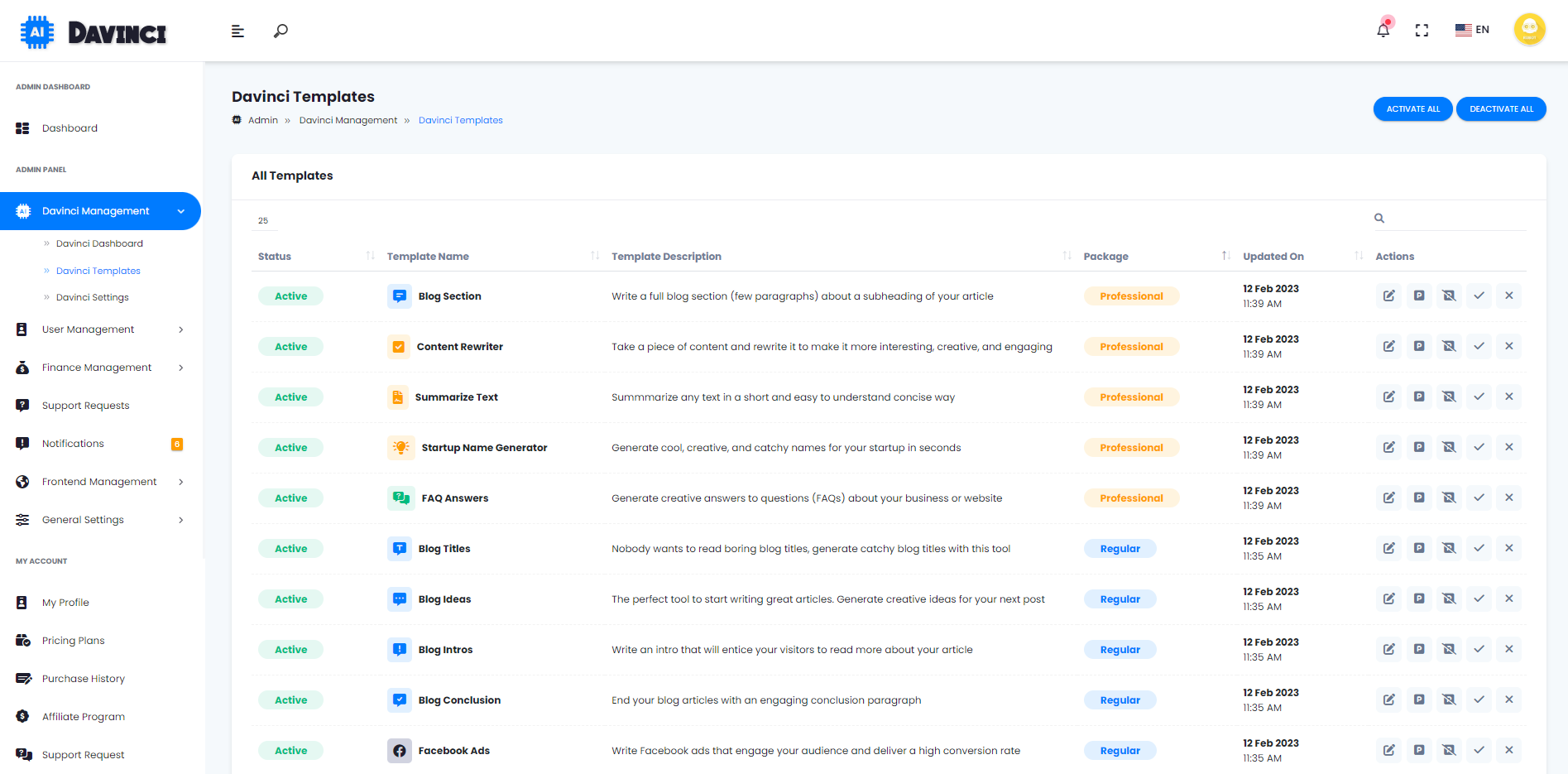This image is a detailed screenshot of the DaVinci AI website, showcasing its user interface and features. The background is predominantly white, providing a clean and professional look. The logo of DaVinci AI is prominently displayed in the top left corner, consisting of the word "DaVinci" in black text. Adjacent to the logo is a small, blue computer chip icon with the letters "AI" in white, emphasizing the site's focus on artificial intelligence.

On the left-hand side of the screen, a vertical navigation menu lists various sections of the website, including options such as "Admin Dashboard," "Admin Panel," and "My Account." These options allow users to manage different aspects of their DaVinci account, including AI-generated articles.

The central portion of the screen features the heading "DaVinci Templates" in bold black text at the top. Beneath this heading, a variety of templates are presented in organized rows. These templates are designed to facilitate the creation of content for websites and blogs and are labeled with names like "Blog Section," "Summarized Text," "FAQ Answers," and "Blog Ideas." Each template includes a brief description; for example, the "Blog Titles" template states: "Nobody wants to read boring blog titles. Generate catchy blog titles with this tool."

On the right side of the screen, each template is accompanied by additional details, including its package type (either "Professional" or "Regular"), the last update date (all listed as February 12, 2023), and action buttons for managing the selected templates.

Overall, the screenshot provides a comprehensive view of the DaVinci AI website's functionality, highlighting its extensive use of templates to generate tailored content for various purposes.